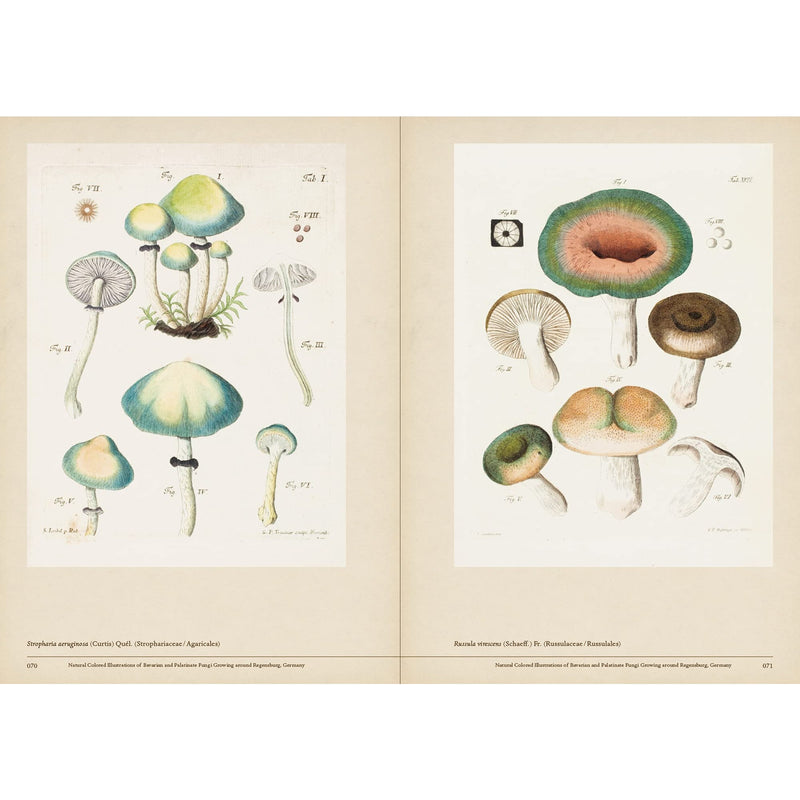This detailed botanical illustration features an open book displaying two pages of meticulously drawn mushrooms against a light tan background. On the left page, there are intricate depictions of green mushrooms with yellow accents, offering a vibrant contrast. The right page showcases a variety of mushrooms in hues of green, brown, and orange. These illustrations are presented from multiple perspectives, including top-down views and cross-sections revealing the gilled undersides. Although there is text accompanying these illustrations, it is rendered in a small font that is not easily readable, adding an element of authenticity to this vintage botanical reference.